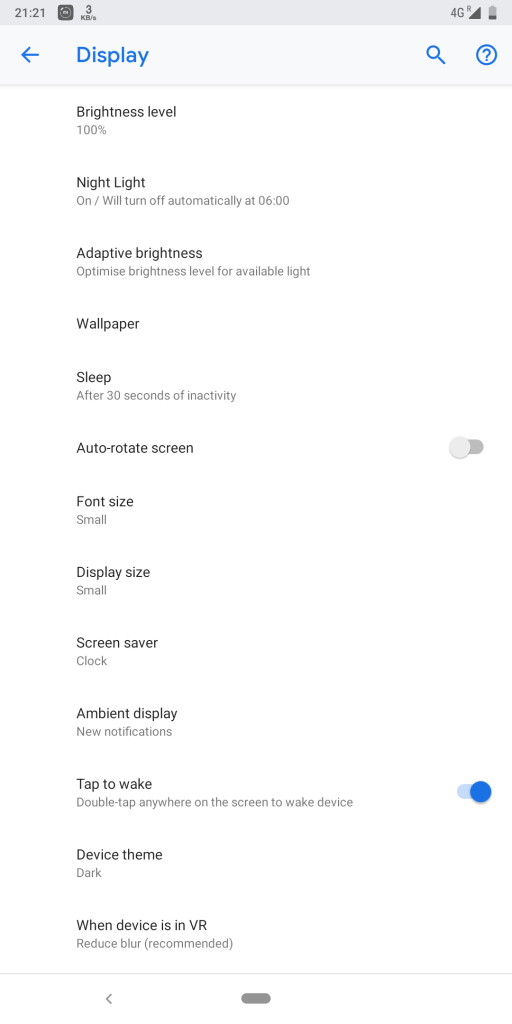The screenshot from the mobile screen displays an array of information and settings in a structured format. At the very top left of the screen, the current time is shown as "21:21". Next to the time is an unidentifiable icon—a black square with an indistinguishable white design—and another icon indicating the number "3" on top of some unreadable text. Moving to the right side of the bar, there is a substantial gap followed by the "4G" network status, a full signal indicator, and a nearly depleted battery icon. All these icons are rendered in dark gray on a lighter gray background.

Below this top bar is a rectangular section with a lighter gray background. This section contains blue icons and text: a left-pointing arrow on the left, the word "Display" in blue text, a search icon, and a circle enclosing a question mark.

The primary section of the screen, appearing below this header, contains the main content on an even lighter gray or almost white background. The content begins with a slider showing the brightness level set at 100% and mentions that "Nightlight" is on, scheduled to turn off automatically at 6 AM. Following this, there are approximately ten more options, including an auto-rotate screen toggle, which is currently off, and a "Tap to wake" feature, which is enabled.

At the very bottom of the screen, a thin, barely noticeable one-pixel line separates the settings options from the phone's navigation UI. This UI contains a left-pointing arrow on the left and a gray oval symbol in the center.

Overall, the image is a detailed snapshot of the settings interface on a mobile device.